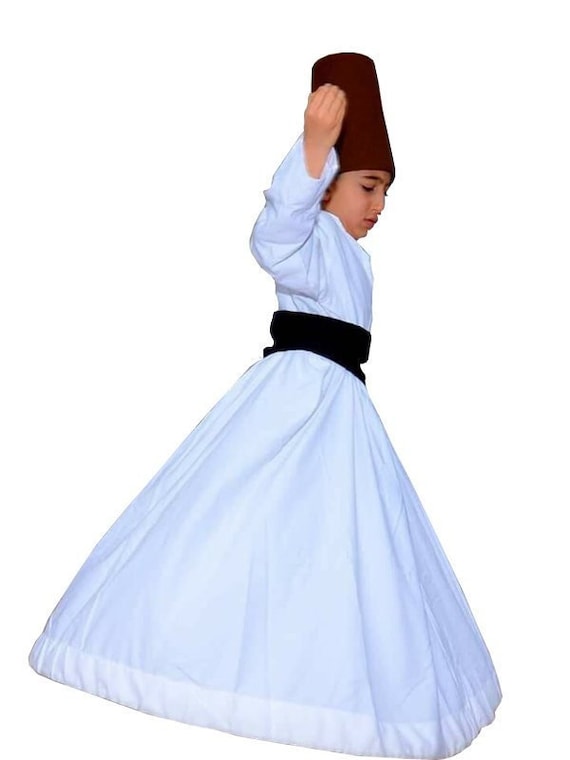The image depicts a young child, seen in a three-quarters view against a stark white background, emphasizing their attire. The child is clad in a long-sleeved, heavy white dress that billows out from the waist into a triangular, almost square shape at the bottom, obscuring their legs and feet. A bright white border trims the hem of the dress, adding contrast to the fabric's thick material. Around their middle is a thick black belt, sash, or girdle, cinching the waist and creating a sharp division between the upper and lower parts of the dress. The child’s right hand is slightly raised, fingers together, positioned near their head, giving an impression of a dance or a poised gesture. Atop the child’s head sits a tall, cylindrical hat, evocative of a Moroccan fez but notably taller, extending upwards in a striking manner. This careful composition, devoid of any other context, directs all attention to the child’s detailed, distinctive outfit and their subtly expressive pose.